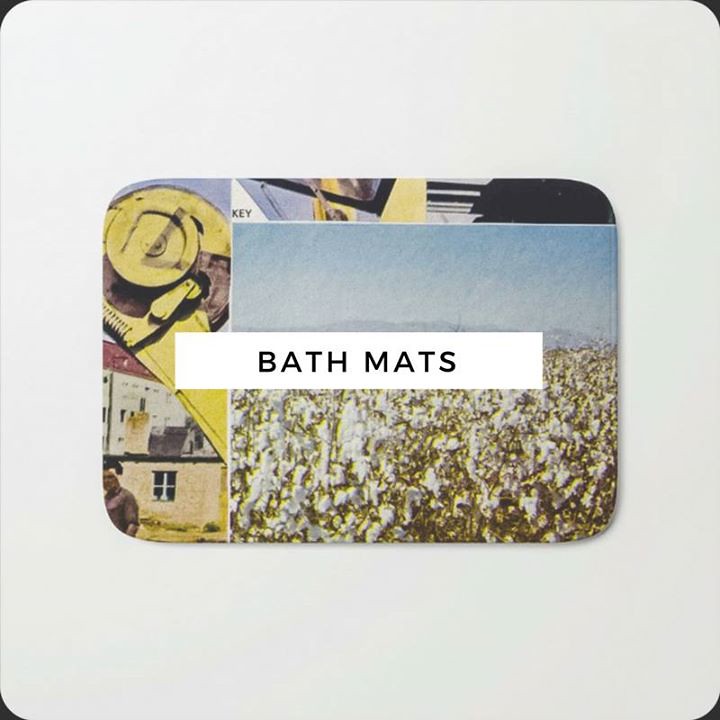This photograph showcases a rounded rectangular bath mat set against a white floor, framed by a white border with small black nicks at each corner, accentuating its roundness. The bath mat features a central white label prominently displaying the words "bath mats" in bold black print. The design on the bath mat is elaborate: occupying approximately 75% from the left and stretching a few inches downward, there is a vast, vibrant green field dotted with large, white flowers beneath a hazy blue sky. Located on the far right side of the mat, a small section depicts yellow construction machinery, possibly a hoe, set against a backdrop of buildings—a tan one in the foreground and a white house with a red roof behind it. A tiny person can be seen in the bottom right corner, adding a touch of human scale to the scene.